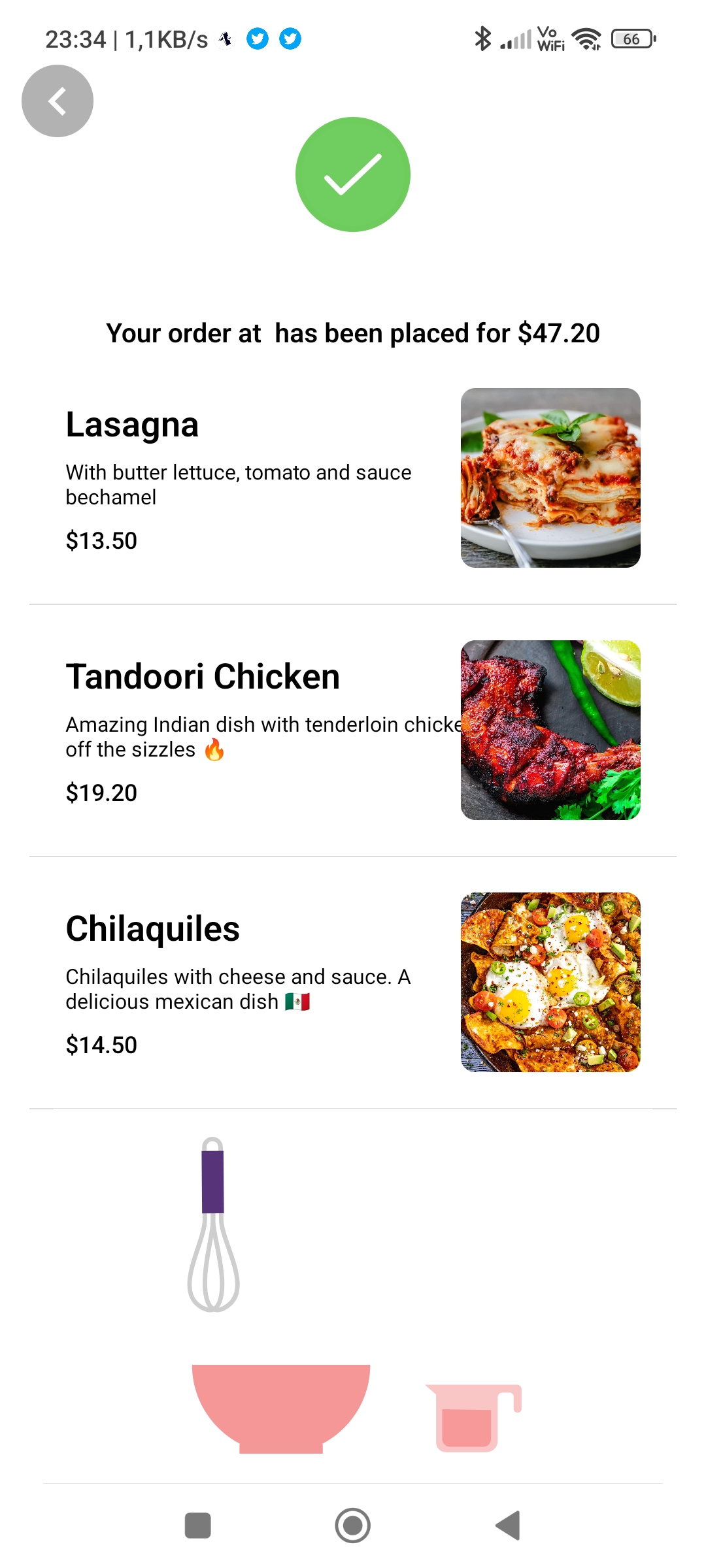This screenshot from an unknown food delivery service app features a confirmation message highlighted by a white checkmark in a green circle, indicating that the order has been successfully placed for a total of $47.20. 

The detailed breakdown of the order includes three distinct dishes:

1. **Lasagna** – Priced at $13.50, this dish is described as featuring butter lettuce, tomato, and a classic bechamel sauce. The image showcases a serving of lasagna on a plate, accompanied by a fork.

2. **Tandoori Chicken** – An exquisite Indian dish, costing $19.20, made with tenderloin chicken. It’s presented alongside some greens and a lime, emphasized with a fire emoji to indicate its spiciness.

3. **Chilaquiles** – Priced at $14.50, this traditional Mexican dish is served with cheese and sauce, accompanied by the Mexican flag emoji. The image includes chilaquiles garnished with eggs.

At the bottom of the screenshot, there’s an illustration depicting a whisk over a pink mixing bowl, with a pink measuring cup filled with liquid, adding a touch of culinary charm to the scene.